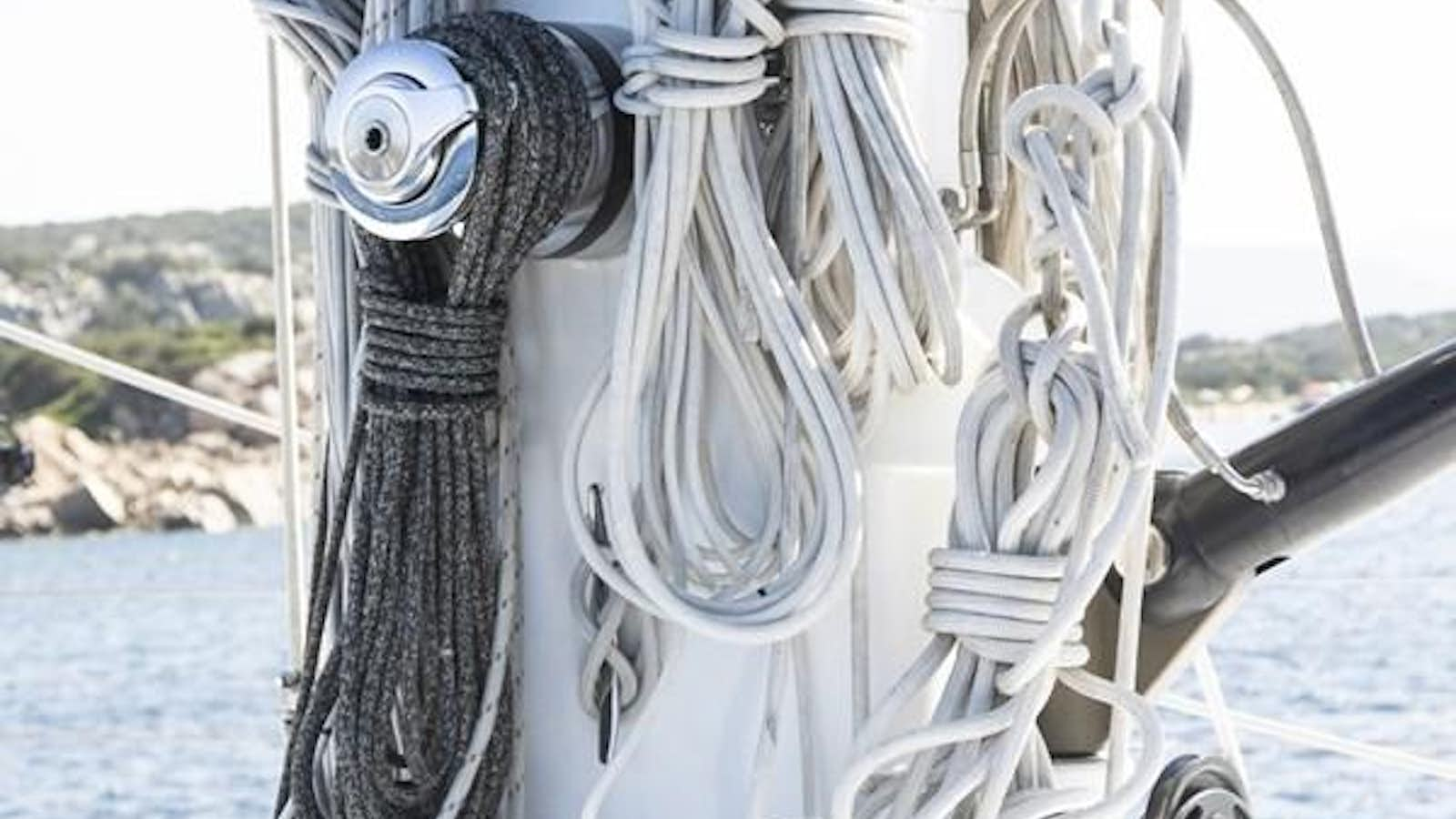A modern boat is depicted with a white-painted plastic mast at its center, adorned with an array of neatly organized ropes. These ropes, mostly white with a gray one among them, are intricately threaded and coiled, then secured to the mast using a shiny silver circular fixture. Additionally, a black metal post with a hinge and a sizable silver bolt is visible to the right of the mast, resembling a fishing pole holder. The backdrop features a tranquil bluish sea with no waves, and a distant rocky shoreline dotted with green foliage, appearing blurry. The left side of the image reveals a white rocky area with patches of green vegetation under a cloudy, white sky. On the right, a similar blurred rocky and green landscape suggests the presence of small, indistinct houses.